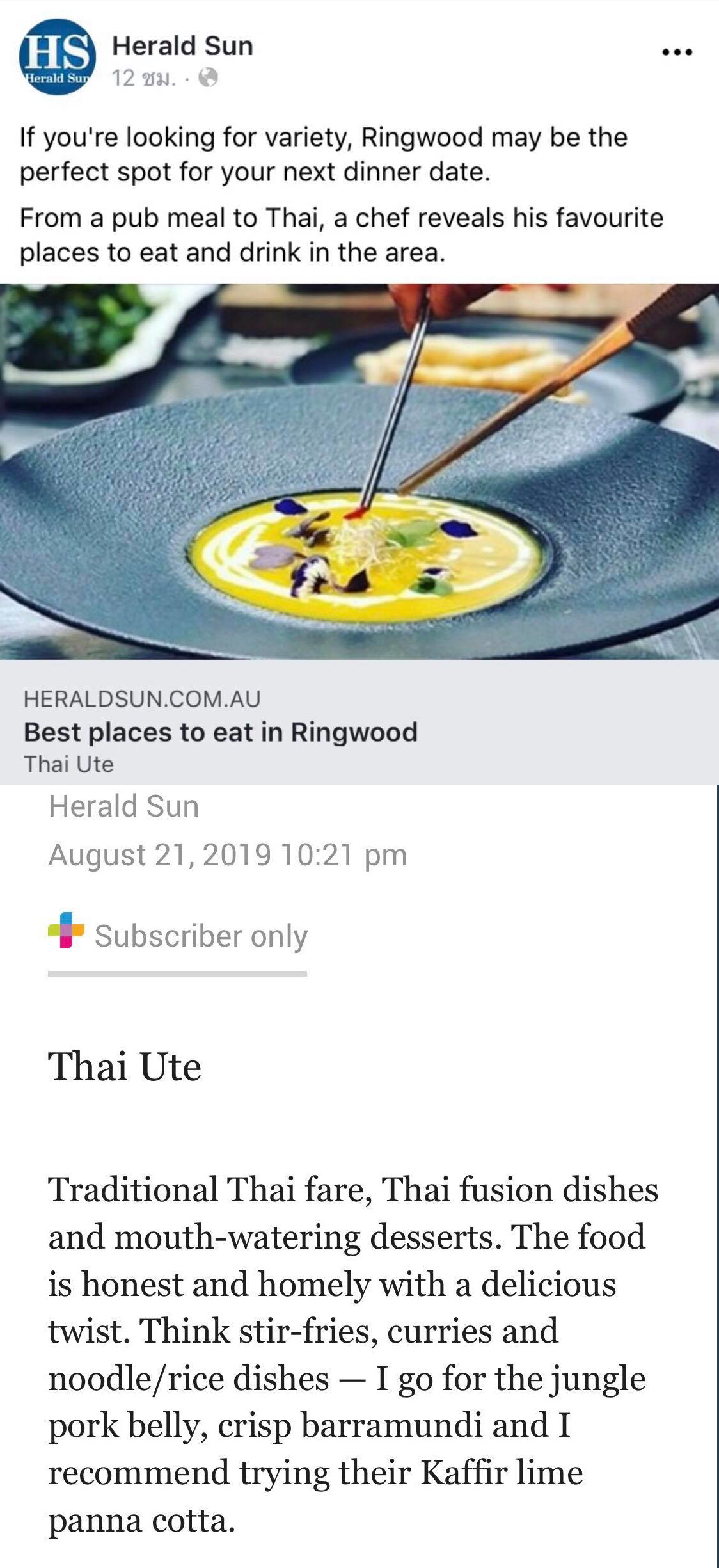This is a screenshot from a mobile phone application. The background starts with a white section in the top left corner, displaying a logo for a website. The logo consists of a blue circle with a white "HS" in it. To its left, in gray font, the number "12" is displayed, accompanied by a globe icon.

Directly below the logo, in black font, there's an informative text stating, "If you're looking for variety, Ringwood may be the perfect spot for your next dinner date. From a pub meal to Thai, a chef reveals his favorite places to eat and drink in the area."

Beneath this text, there's an aesthetically presented photograph of a wok, showcasing someone's hand using chopsticks to mix egg yolk with cheese and other ingredients, attempting to create an artistic impression.

Following the image, there's a gray rectangle containing text in black font. Below this rectangle, the timestamp "10:21 PM" is shown in gray font on a white background, along with the note "subscriber only." Further down, additional text in black font is visible, though the content of this text is not specified in the provided description.